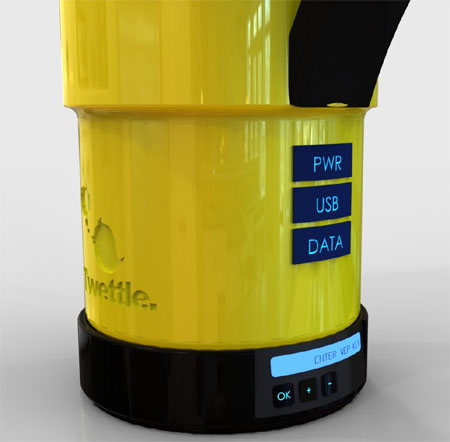The image features a black and yellow cylindrical flashlight with a wide mouth, positioned centrally against a solid background that transitions from a light gray at the top to a darker shade at the bottom. The majority of the flashlight is yellow with several distinct sections. The base is round and black, featuring three blue-labeled buttons: "OK," "Plus," and "Minus." Above these buttons, there is a white label that says "Enter WEP."

The left side of the flashlight displays the brand name "TWETTLE," accompanied by a logo of a bird with a thought bubble. On the right side, there are three stacked blue rectangles with white text: "PWR" at the top, "USB" in the middle, and "DATA" at the bottom. The top portion of the flashlight, also yellow, has a black handle protruding to the right, and the uppermost part of the flashlight is not visible as it is cut off by the frame of the image. The object is described as a tool or appliance, suitable for various settings such as a workplace, store, or home due to its functional design and labeled features.